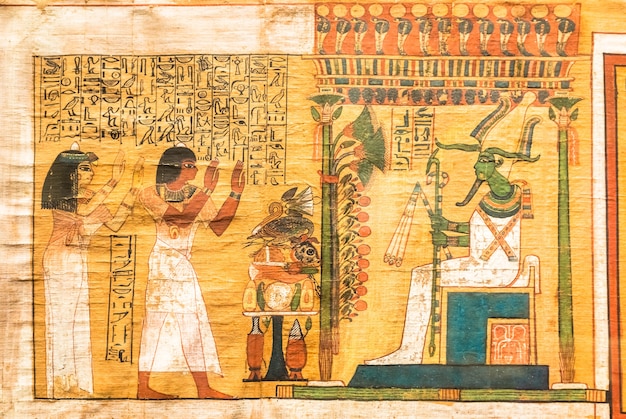The image depicts an aged and worn Egyptian painting with a distinct landscape orientation. On the left side, there's an Egyptian woman and man, both clad in long white tunics and featuring black hair. The man wears a black necklace and cuff bracelets. Their hands are raised, as if in a gesture of worship. Between them and the deity is a vertical column of hieroglyphics, with numerous additional columns of hieroglyphics above their heads. 

To their right is a throne, painted in a blue hue. Sitting on this throne is a green-skinned deity with long green hair and possibly a beard. This figure is adorned in a white bodysuit and a yellow or gold headpiece, holding a tall green cane in one hand and a rod with a white fan in the other. Behind the deity, more green poles or columns can be seen. The background of the entire scene is a tan cream color, and shelves with various items occupy the space between the worshippers and the deity. The piece is vibrant with numerous Egyptian symbols and bright colors, adding to its rich detail and historical ambiance.